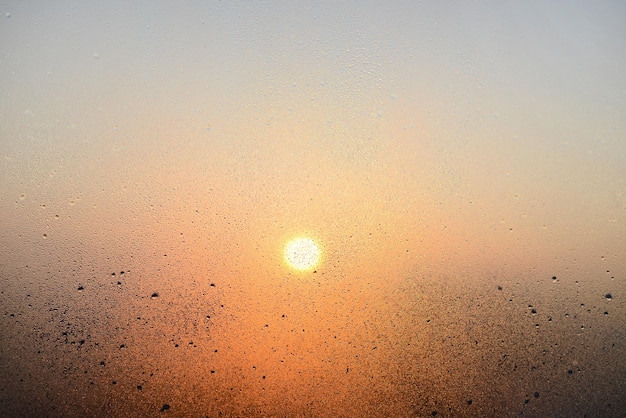This image captures a scene of the sun viewed through a window, creating a distinctive and somewhat artistic impression. The bright yellow ball of the sun, encircled by an orange halo, is centrally positioned against a backdrop of a cloudy, grey sky. The sun appears slightly blurred and distorted due to the window, enhancing the artistic effect.

In the lower part of the image, there is a striking gradient, shifting from grey in the upper part to deep orange near the bottom. The bottom corners of the frame feature dark grey splotches, almost forming a vignette that directs attention towards the central sun. 

The scene is further enriched by droplets of liquid scattered across the window's surface, particularly concentrated in the bottom third of the frame. Each droplet, along with numerous grey dots, is illuminated along its bottom edge and casts a dark shadow on the top, creating a dynamic interplay of light and shadow. This combination of elements—blurred sunlight, varying colors, and abstract droplet patterns—gives the image a unique, almost painted aesthetic, resembling an abstract art piece or perhaps a view through a dewy car windshield at sunrise or sunset.